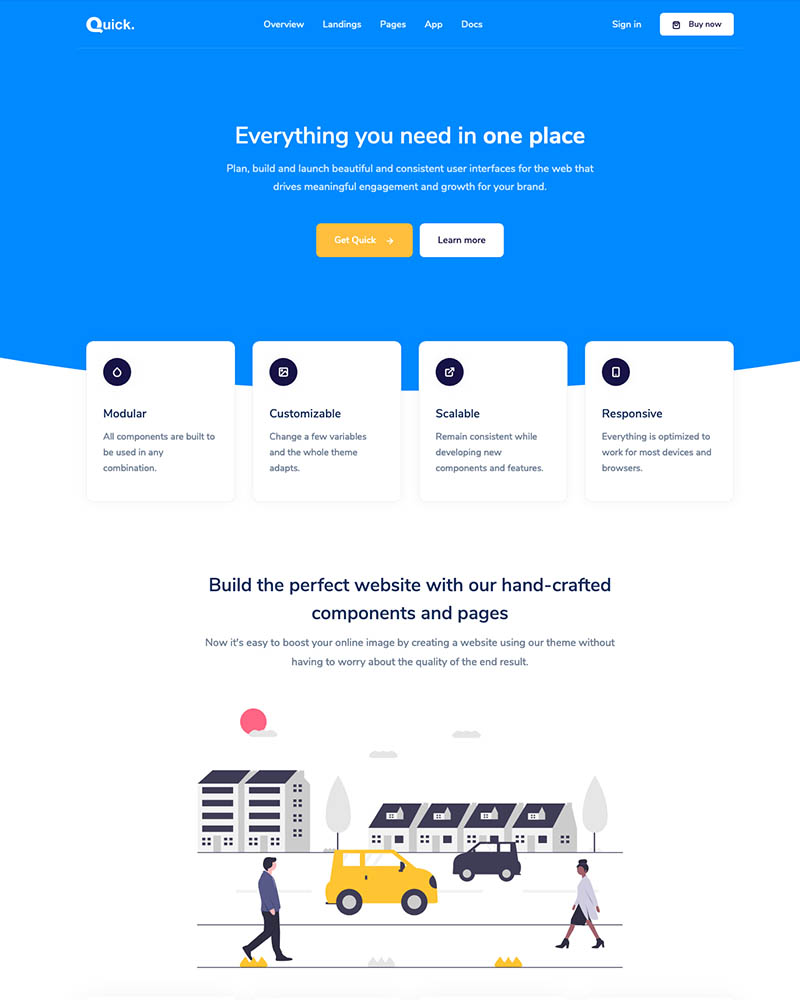Here is the cleaned-up and detailed caption for the image:

The image is a polished screenshot of a website named "Quick", highlighted by a distinct blue border at the top. The site name, "Quick," is prominently displayed in white font, followed by a period. To the right of the site name, the navigation menu includes options: "Overview", "Landings", "Pages", "Apps", and "Docs". On the far right, there are "Sign In" and "Buy Now" buttons, the latter styled as a white button.

Just below the top border, the website headline reads, "Everything you need in one place, plan, build, and launch." It promotes the creation of beautiful and consistent user interfaces for the web, meant to drive meaningful engagement and growth for your brand. Two prominent buttons are featured: "Get Quick" in a vibrant yellow and "Learn More" in white.

Further down, the features of the service are distilled into four main points, each within a white square box and described in navy blue text:
1. **Modular**: All components are built to be used in any combination.
2. **Customizable**: Change a few variables and the whole theme adapts.
3. **Scalable**: Remain consistent while developing new components and features.
4. **Responsive**: Everything is optimized to work with most devices and browsers.

A descriptive line encourages users to build the perfect website with Quick's handcrafted components and pages, emphasizing the ease of boosting one's online presence without compromising quality.

At the bottom of the screenshot, there is a cartoon illustration of a man and a woman walking towards each other on a sidewalk, accompanied by a yellow and blue car driving down a road, adding a touch of animation and friendliness to the overall design.